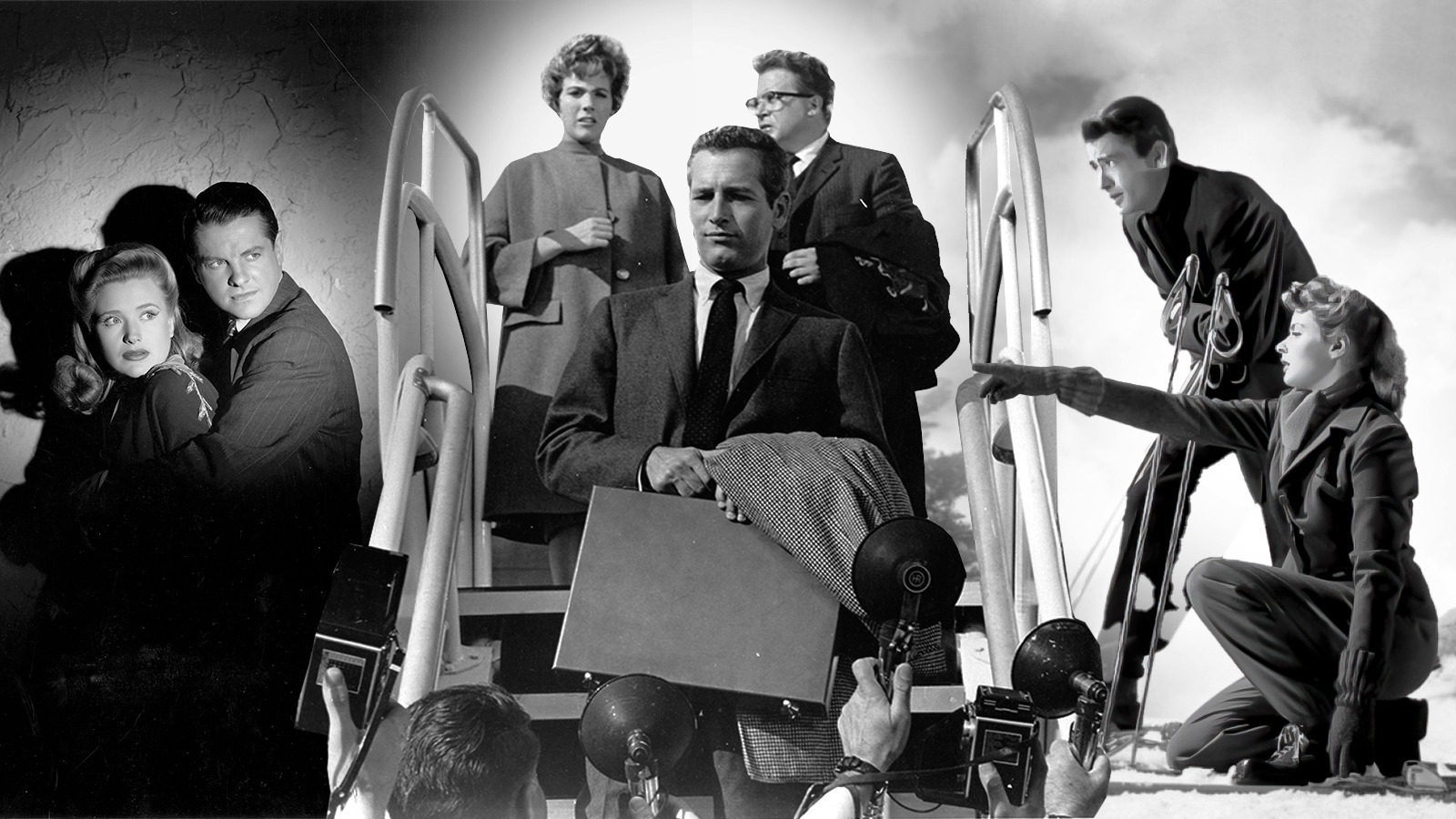A black and white triptych of scenes from what appear to be classic films, each evoking a dramatic moment of intense emotion. 

On the left, a distressed man and woman are huddled together, their expressions conveying fear and uncertainty. They are illuminated by a stark light, which casts deep shadows against a textured background, heightening the sense of foreboding.

In the central panel, a trio of individuals are seen descending a staircase: a man carrying a suitcase, dressed in a shirt, another man, and a woman. Their weary, downtrodden demeanors suggest a moment of despair or confrontation, as they engage with a solitary figure at the base of the stairs.

The rightmost scene captures a man and woman in a moment of tension. The man is gripping a metal object that resembles a trombone, while the woman kneels on the ground, pointing toward something out of frame to the left. Above them, a moody, cloud-filled sky adds an ominous tone to the tableau.